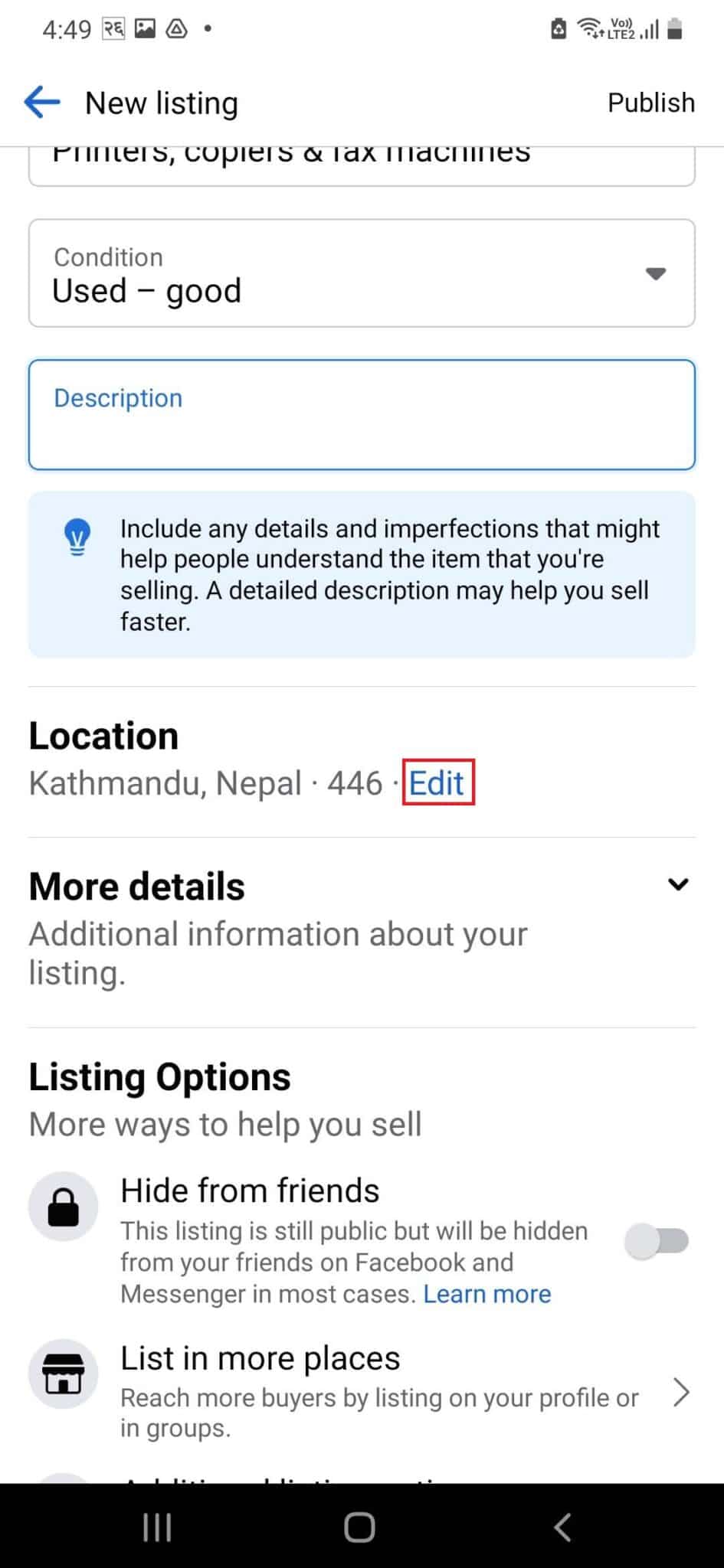This is a detailed caption for the image described:

---

**Screenshot of Facebook Marketplace New Listing Interface on a Samsung Smartphone**

The image captures a screenshot taken on a Samsung smartphone, displaying the Facebook Marketplace new listing interface within the Facebook app. The overall background of the screenshot is white.

**Top Bar:**
- The very top bar shows various icons including:
  - Time (positioned to the far left)
  - Screenshot icon
  - Google Drive icon
  - Wi-Fi icon
  - Mobile data icon
  - Battery saver icon
  - Battery icon (indicating the remaining battery percentage)

**Main Content:**
- The main content area is dedicated to creating a new listing on Facebook Marketplace.
  - At the very top left corner, the text "New Listing" is prominently displayed.
  - To the right of "New Listing," there is a "Publish" button.
- Below this, several horizontal text boxes and options are visible:
  - The first text box displays a category, partially visible as "Printers, Copiers, and Fax Machines."
  - The second option specifies the item's condition, which is selected as "Used - Good."
  - Following this is a description box outlined in blue, with an instructional text box underneath it in light blue. The text reads: "Include any details and imperfections that might help people understand the item that you're selling. A detailed description may help you sell faster."
- Further down, the current location is shown in bold as "Kathmandu, Nepal," with the option to edit this location outlined by a red square.
- There is a "More Details" section that expands to provide additional information about the listing.
- Towards the bottom, under "Listing Options," users are given more ways to enhance their listing:
  - "Hide from friends," which is toggled off.
  - "List in more places," indicating the option to list in different groups on Facebook Marketplace.

This structured and detailed view effectively guides the user through the process of creating and optimizing a new listing on Facebook Marketplace.